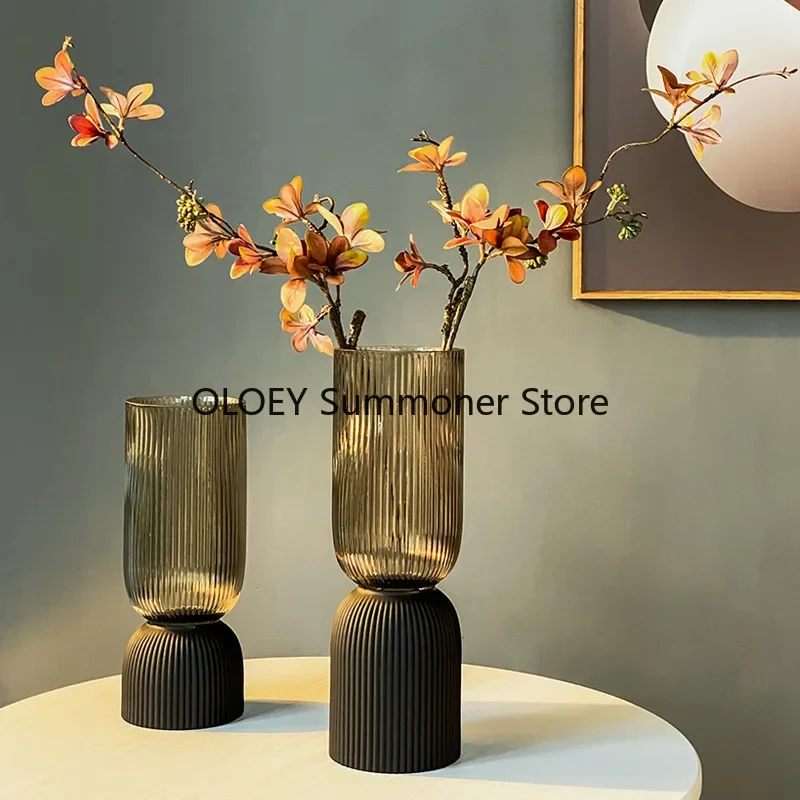In this image, two uniquely designed glass vases sit on a white circular table against a grey backdrop. The vases, featuring intricate vertical lines, are partially see-through when hit by light. The taller vase, positioned on the right, houses two orange-red flowers with twig-like stems. These flowers, while vividly colored, have a slightly artificial appearance. The vase's top half is translucent, obstructed by its decorative lines, while the bottom is black. The shorter vase to the left remains empty, showcasing its light grey and somewhat transparent structure. In the top right corner of the image, a dark-framed picture is partially visible, displaying a black background with a white object that could resemble an egg. Overall, the scene is bathed in a subtle light that emphasizes the textures and colors of the vases and flowers.